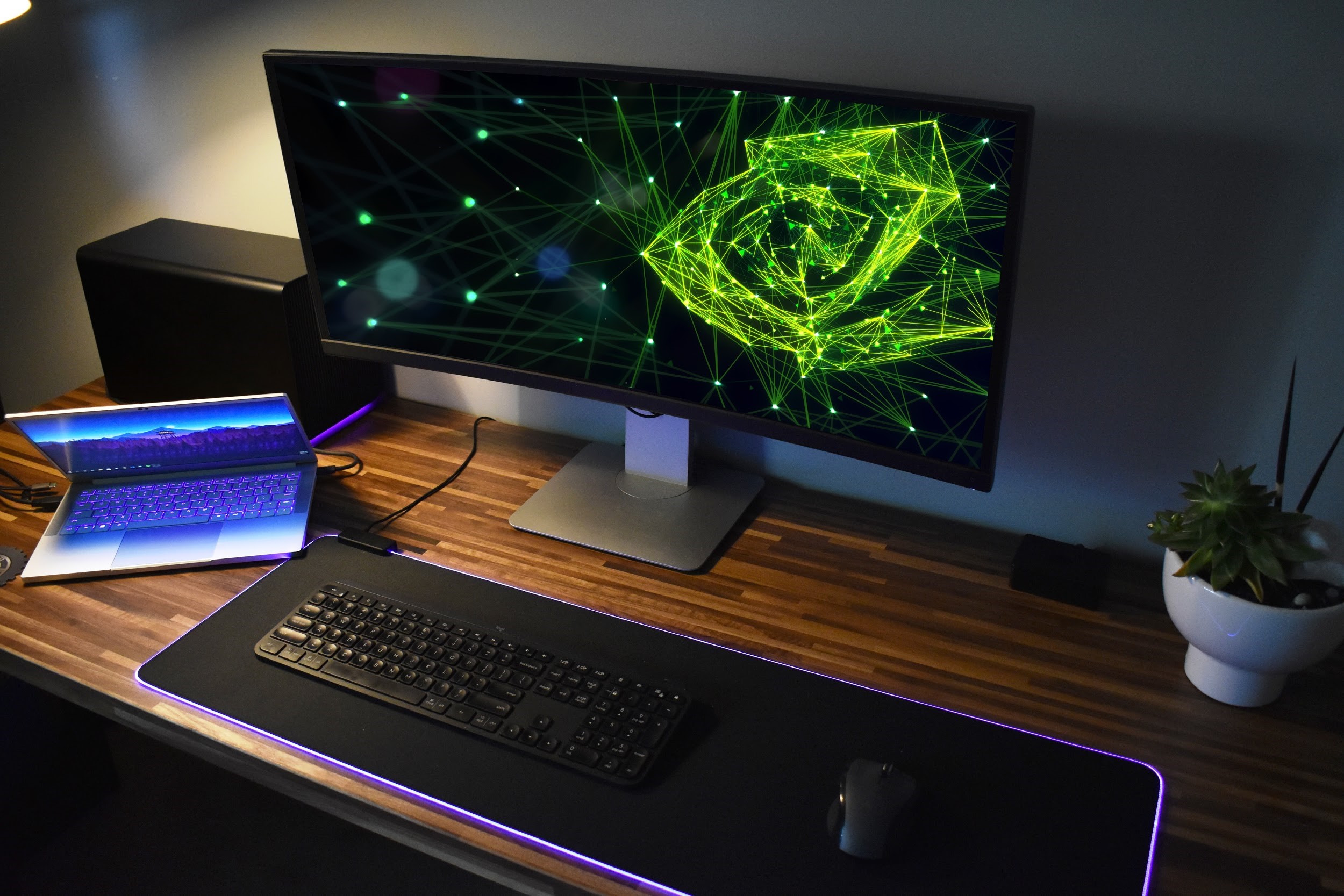In this detailed image of a personal computer setup, the scene unfolds on a sophisticated wooden desk featuring thin slats. Centered prominently is a large, modern curved LCD monitor displaying an abstract geometric screensaver with bright yellow connecting lines, reminiscent of spotlights. Adjacent to the monitor on the right sits a sleek black keyboard with a blue outer lighting edge, accompanied by a black mouse on a stylish pad. To the left, a partially opened silver laptop showcases a picturesque mountain scape on its screen. Further left sits the PC tower—an essential component of this advanced setup. Adding a touch of nature, a white porcelain pot holding a vibrant green succulent is positioned at the middle right of the desk. The entire arrangement rests against a blue-gray wall, suggesting an indoor setting likely within a bedroom. The harmonious blend of neon green, purple, blue, mahogany, gray, and black accents creates a visually stimulating and modern workspace.